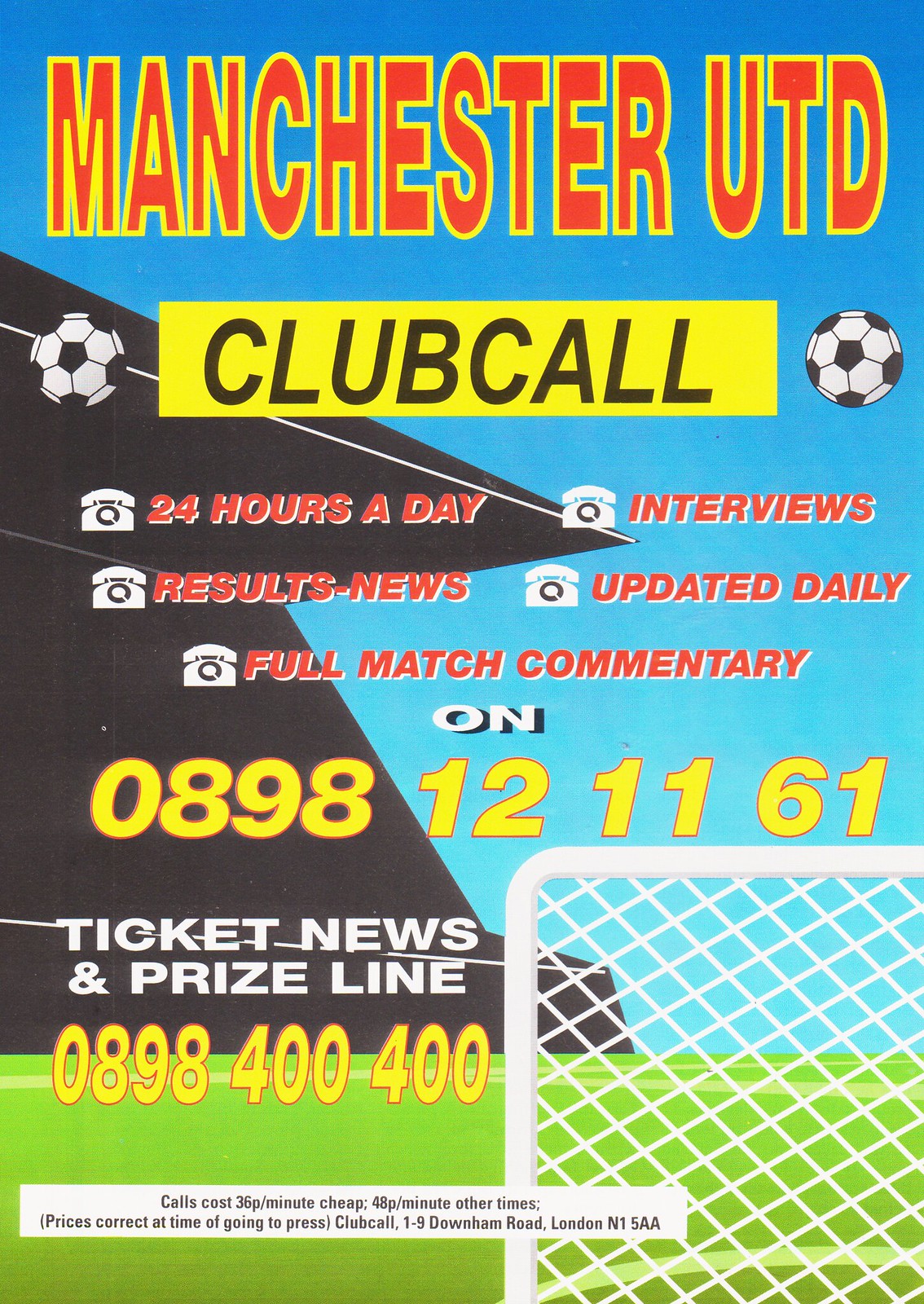The advertisement poster for the Manchester United Call Club features a vibrant and detailed cartoon-style illustration with a blue sky background, a black stadium structure with white lines, and a green football field with a white goal net. At the top, bold red letters outlined in yellow spell out "MANCHESTER UTD." Below, within a yellow rectangle, "CLUB CALL" is prominently displayed in black capital letters, flanked by black and white soccer balls on either side.

The poster highlights five key services provided by the call club, each indicated by a white telephone icon accompanied by red text reading "24 hours a day," "interviews," "results-news," "updated daily," and "full match commentary." Beneath these services, the word "ON" appears in white, followed by a yellow font featuring the primary call number "0898 121161." Below this, the poster provides additional contact information for ticket news and prize line, displayed in white and yellow font respectively: "TICKET NEWS and PRIZELINE" with the number "0898 400400."

A disclaimer at the bottom of the advertisement, in black text on a white background, informs callers that calls cost 36 pence per minute during cheaper periods and 48 pence per minute at other times, noting that these prices were correct at the time of publication. It also lists the address for Club Call as "1-9 Downham Road, London N1 5AA." This advertisement clearly serves as an engaging flyer to encourage fans to dial into the Manchester United Call Club for the latest updates and interactive experiences related to the football club.